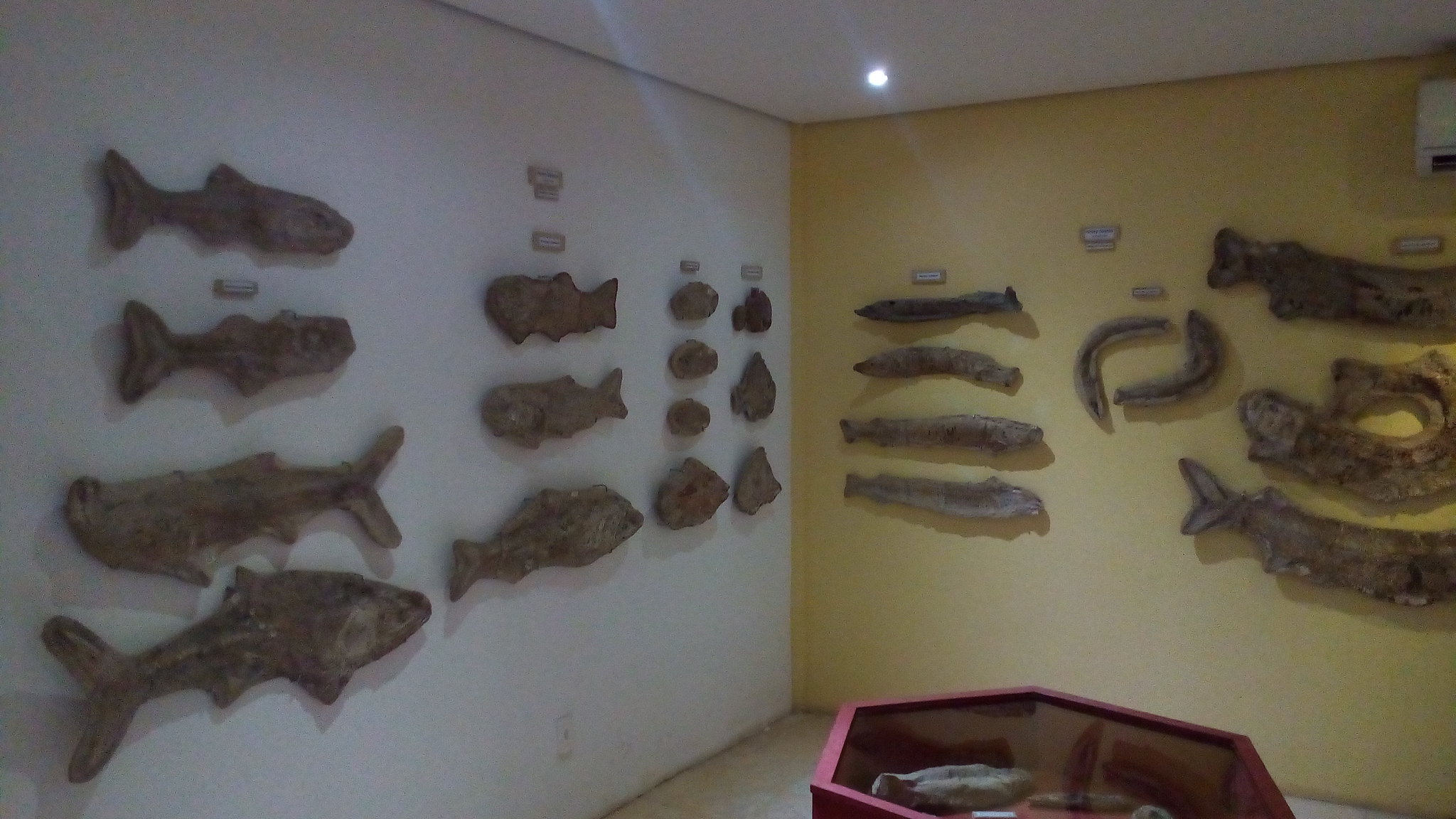This photograph captures a dimly-lit corner of a room where two walls meet, adorned with numerous wooden fish carvings. The left wall, painted white, and the right wall, a faded yellow, create a stark contrast in the corner. 

On the white wall, a series of brown wooden fish carvings are arranged in a meticulous pattern. Starting from the far left, there is a vertical row of four fish with alternating directions; the top two face right, the middle one faces left, and the bottom one faces right. Adjacent to this row, another vertical arrangement showcases three fish, with the top two facing left and the bottom one facing right. Further to the right, there are two more rows of four fish, though they are harder to discern clearly in the dim lighting.

The yellow wall features additional fish carvings, seemingly larger and more spaced out. Near the corner, a vertical row of four fish is arranged from top to bottom. Next to it, two fish are positioned in the middle of the wall, resembling boomerangs, facing opposite directions. To the far right, three large fish are placed vertically, with similar alternating directions and the middle fish’s tail curling above its body, partially extending out of the photograph's frame.

In the bottom right corner, a glass-covered display case with a red hexagonal wooden frame contains more fish carvings, though the details and labels within the case are not clearly visible due to the photograph’s poor clarity. The ceiling, painted white, completes the framing of this corner scene, adding a subtle contrast to the overall muted color palette.